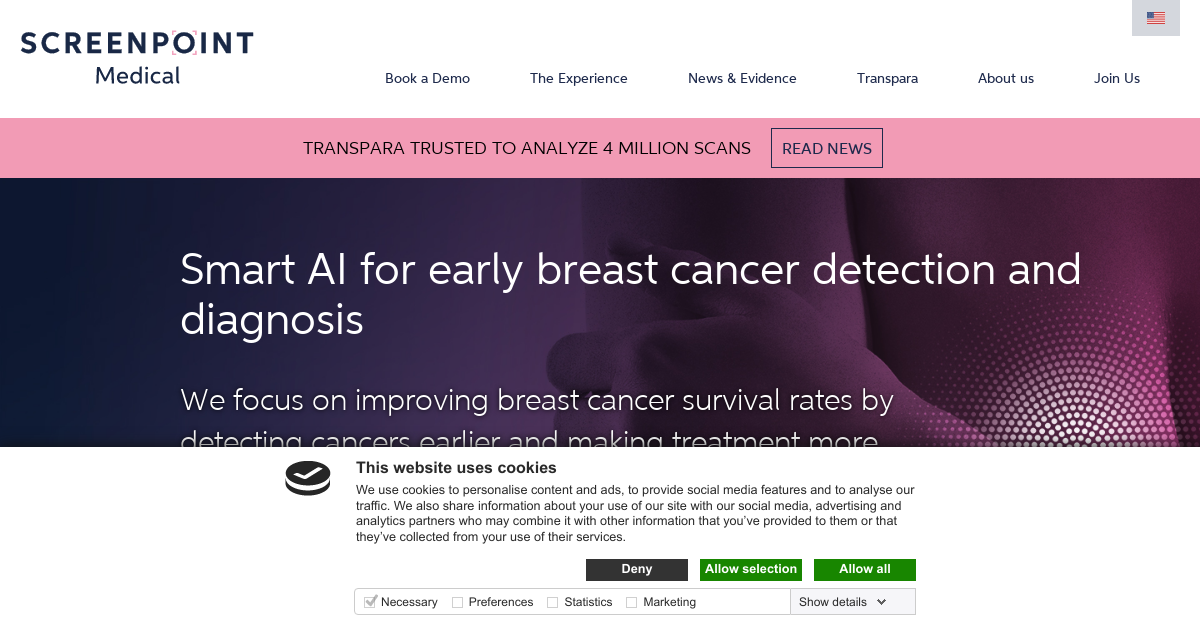This is a screenshot of the ScreenPoint Medical website as viewed on a desktop browser. The top of the page features a white header bar with the ScreenPoint Medical logo on the left. The logo is stylized with "ScreenPoint" in a larger font above the word "Medical," and "Medical Center" is highlighted in purple beneath it. 

Near the middle of the header bar, there are several navigational options: "Book a Demo," "The Experience," "News and Evidence," "Transparency," "About Us," and "Join Us." On the top right, you can select your language, indicated by an American flag inside a gray box directly above the "Join Us" option.

Directly beneath the white header is an eye-catching pink bar, apparently designed to look urgent, resembling a "Breaking News" ticker. This banner reads: "Transparency. Trusted to analyze four million scans. Read news."

Below this urgent banner, the main section of the website begins. It prominently features a background with abstract purple shapes. The primary call to action is prominently displayed: "Smart AI for Early Breast Cancer Detection and Diagnosis," emphasizing a focus on improving breast cancer survival rates. 

At the bottom of this section, there is a box for users to accept or deny cookies.